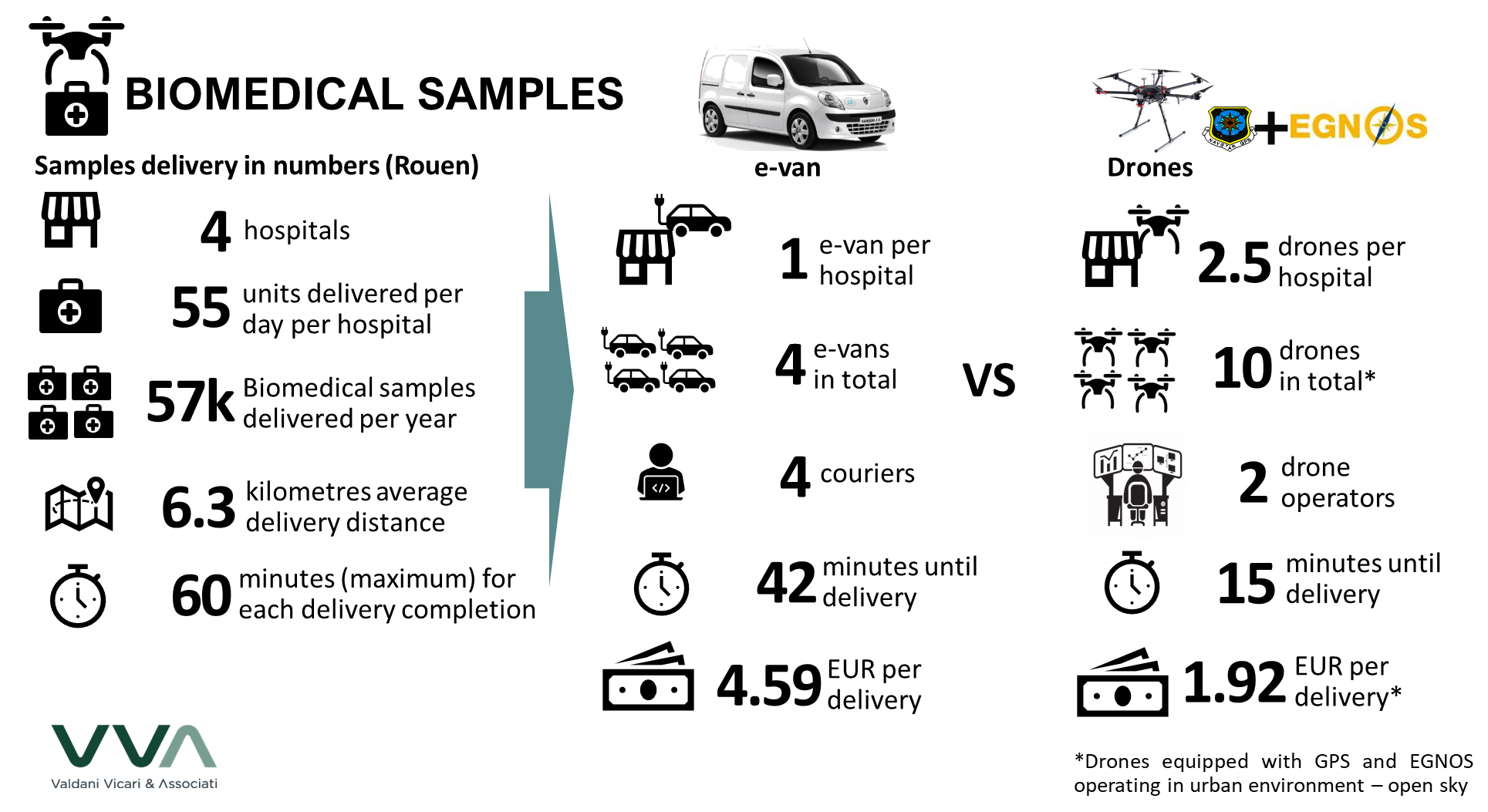The infographic presents a black-and-white comparison between two delivery methods for biomedical samples: traditional e-vans and drones. The background is white with black text, interspersed with some colored icons like a dark gray-green arrow and the colored logo of a helicopter carrying a briefcase with a cross.

At the top left, in large font, it reads "Biomedical Samples." Beneath this, the header "Samples Delivery in Numbers" introduces the data. The left section lists delivery statistics: "Four Hospitals," "55 Units Delivered Per Day Per Hospital," "57K Biomedical Samples Delivered Per Year," and "6.3 Kilometers Average Delivery Distance."

Below these stats, the infographic shifts focus to the comparison, with a "VS" prominently displayed between columns for e-vans and drones. The e-van column features an image of a white van with a black windshield, labeled "E-Van." Details include: 
- "One E-Van Per Hospital" 
- "Four E-Vans in Total"
- "Four Couriers"
- "42 Minutes Until Delivery"
- "4.59 Euros Per Delivery"

The drone column describes alternative stats:
- "2.5 Drones Per Hospital"
- "10 Drones in Total"
- "Two Drone Operators"
- "15 Minutes Until Delivery"
- "1.92 Euros Per Delivery"

At the bottom right, small text reads: "Drones equipped with GPS and EGNOS, operating in urban environment - open sky." The infographic is hosted by Valdani, Vicari, Associati (VVA), likely indicated at the very bottom. This detailed presentation highlights the efficiency and cost-effectiveness differences between e-vans and drone deliveries for biomedical samples.